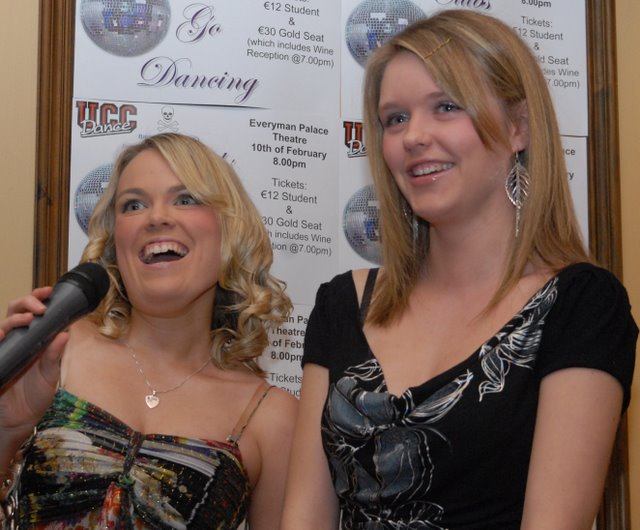The image features two young women, dressed up and standing in front of a white sign associated with the UCC dance event at the Everyman Palace Theater on the 10th of February, advertising tickets at £12 for students and £30 for a gold seat, which includes a wine reception at 7 p.m. The woman on the left, who appears slightly younger, has curly hair just below her shoulders and is wearing a colorful spaghetti strap dress in green, white, red, and black. She’s smiling and holding a microphone, possibly being interviewed. She also wears a gold necklace with a heart pendant. The woman on the right, who seems older, has straight blonde hair of a similar length and is adorned with silver dangling earrings featuring a leaf pattern. She's wearing a black dress with a white floral design and smiling as well. Both women are looking slightly to the left, suggesting they might be involved in officiating or announcing at the dance event. The woman on the left has larger eyebrows and eyes with a more intense expression, while the woman on the right has a softer look.